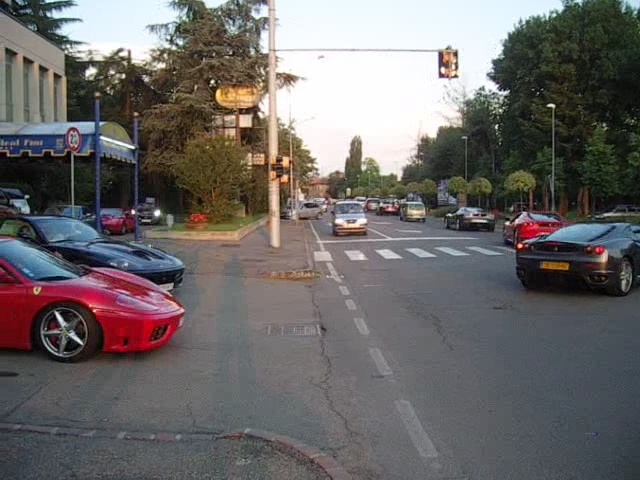This vibrant color snapshot captures a bustling street scene as if viewed from the corner of a busy intersection. The multi-lane road features a blend of direct and angle parking that serves a shopping center parking lot opening onto the street. A traffic stop light presides over the scene, guiding cars traveling in both directions. Prominently, a striking collection of Ferraris is visible: a red Ferrari and a black Ferrari are poised to exit from a driveway on the left, likely leading from a hotel or maybe a Ferrari dealership, denoted by a blue awning under which more Ferraris are parked. In the foreground, a dark gray Ferrari has just pulled into the lane, while farther ahead on the right side of the street, a series of red and gray Ferraris continue down the road. The scene is framed by tall, green trees lining both sides of the street, adding a natural vibrancy to the busy urban environment.